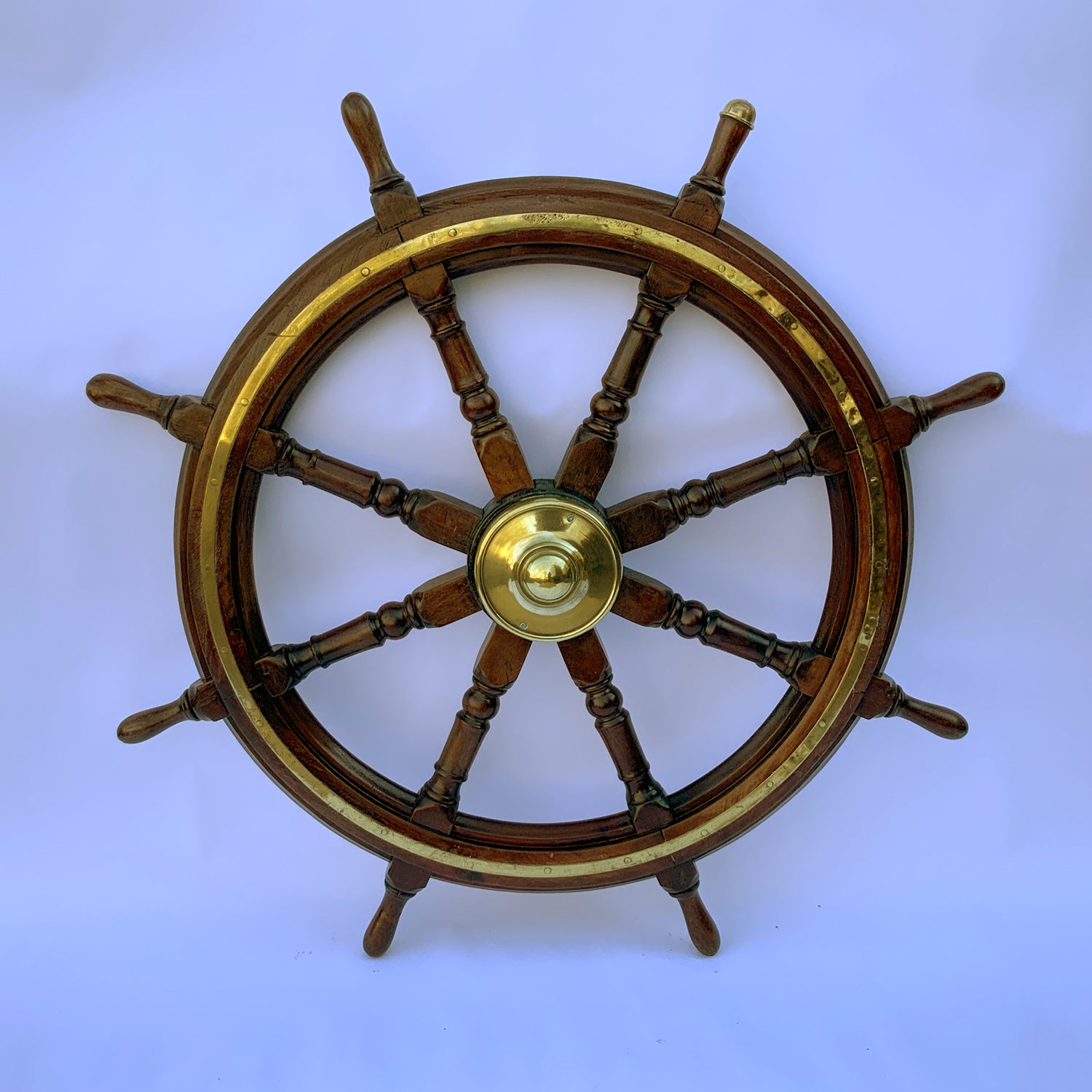The photograph depicts an ornate ship's wheel, constructed from dark brown wood, with a striking gold or brass trim that encircles the rim. The center of the wheel is filled with intricate gold accents, adding an opulent touch to its already distinguished appearance. This wheel features eight protruding handles, with one notably adorned with a gold or brass cap, suggesting its use as a main steering point. The handles and central spokes display elaborate carvings, enhancing the decorative aspect of the wheel. The background is a light baby blue or lilac hue, and the shadows cast to the right side of the wheel indicate that the light source is coming from the left. This historical artifact evokes imagery of ancient ships, potentially displayed in a museum setting, reminiscent of maritime adventures and iconic figures like Captain Jack Sparrow.